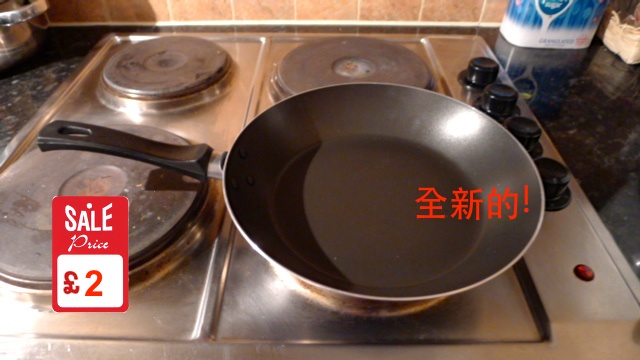This image depicts a close-up view of a kitchen stovetop with four burners. The burners are flat-topped, and three of them are covered with silver metal coverings. On the front right burner, there is an aluminum frying pan that features some red Chinese letters followed by an exclamation mark on its right-hand side. In the lower left-hand corner of the image, a red rectangle with the text "SALE PRICE" in white letters, and "2 Euros" with a red number 2, is visible. The stovetop is set in a black granite countertop, visible in the upper left-hand corner and on the right side of the image. Additionally, the backsplash at the top of the image is composed of brownish-colored tiles. Four control knobs are aligned on the right-hand side of the stove.